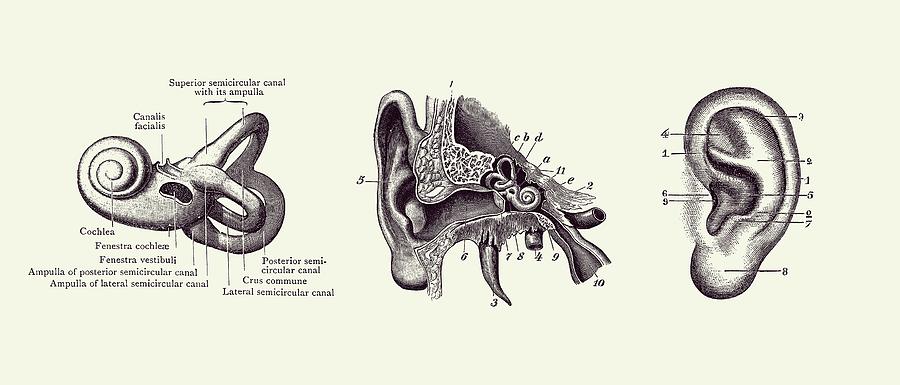This detailed black-and-white hand-drawn diagram illustrates various views of the human ear, spread across three distinct images arranged side by side on a cream-colored background. The rightmost image displays a front-facing view of someone's left ear, meticulously labeled with up to nine numerical callouts highlighting different aspects. Adjacent to this, the middle image presents a detailed sectional view of the ear's internal structure, brimming with arrows and numerical as well as alphabetical callouts, facilitating an understanding of the ear's internal anatomy. The leftmost image delves deeper into the anatomy, showcasing the superior semicircular canal with its ampulla and featuring intricately labeled parts, including a uniquely shaped structure reminiscent of a snail shell that transitions into a 3D object. The shading techniques employed with the pencil add depth and texture to each diagram, enhancing their illustrative clarity.